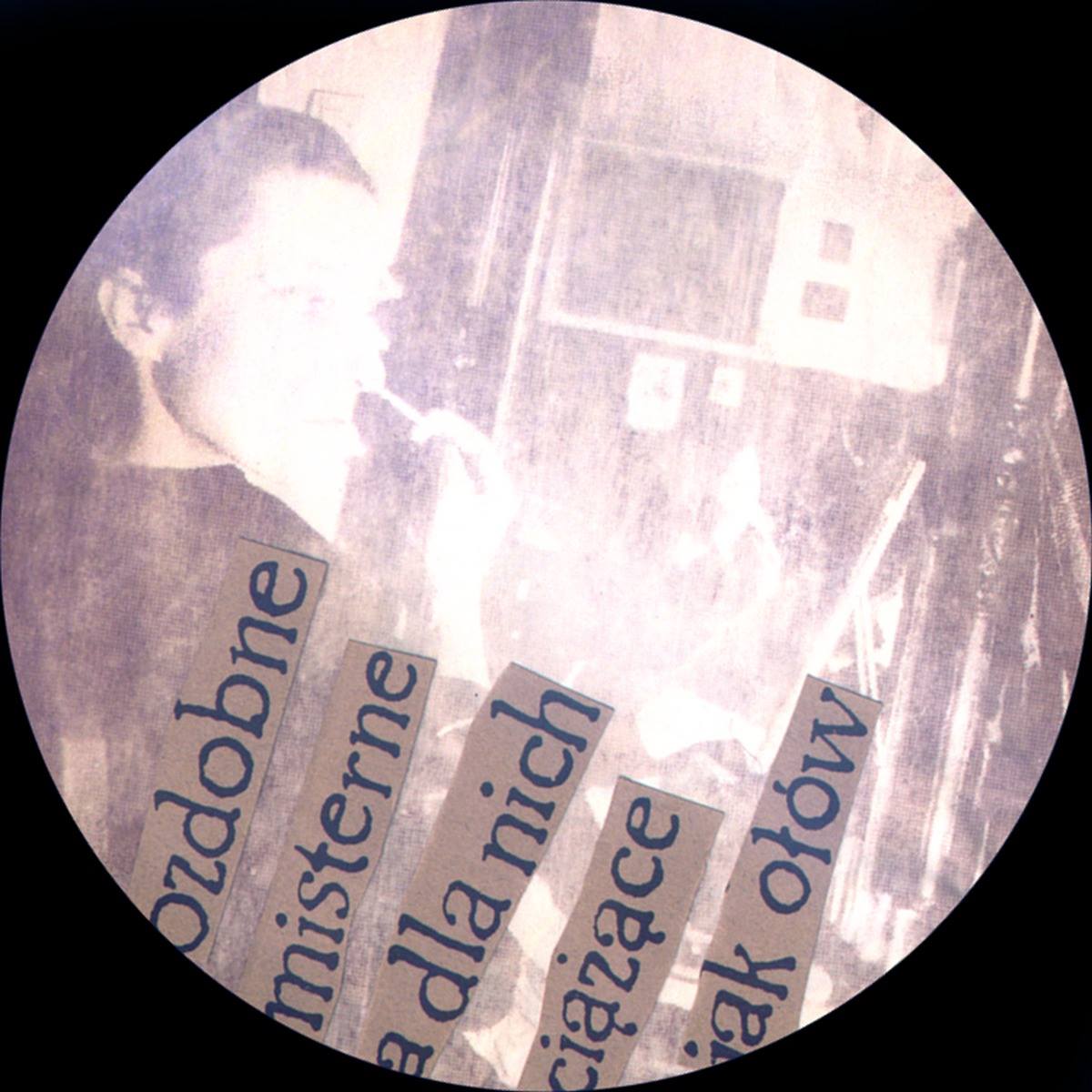The image is an abstract mixed-media piece featuring a large, perfect circle set against a completely black background. Inside the circle is a highly overexposed and grainy, blurred photograph of a person on the left-hand side, facing towards the right. The individual, whose gender is indiscernible, appears to be holding something in their hand and has wide-open eyes. The background within the circle seems to depict fragmentary and indistinct objects, possibly a microwave and a painting easel, which are washed out in faded purple tones. Below the person, at the bottom of the circle, there are five vertical strips of paper with cut-out words in an off-white background. These words appear to be in a different language, possibly German, with letters that spell out, "O-Z-D-O-B-N-E," "M-I-S-T-E-R-N-E," "A-D-L-A-N-I-C-H," "C-I-A-Z-A-C-E," and "I-A-K-O-T-O-W." The overall image is minimal in detail due to its washed-out, blurred effect, and the text adds an additional layer of abstract complexity.